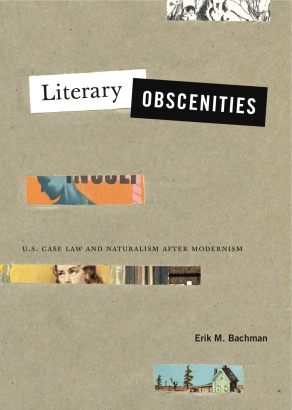The image depicts the cover of a book with a background resembling recycled light brown paper with an olive tint, featuring characteristic speckles. Various cut-out magazine snippets are pasted onto this background. At the top center, two prominent rectangles stand out: the left white rectangle with black text reading "Literary," and the right black rectangle with white text reading "Obscenities," which together form the book's title, "Literary Obscenities."

Below this title, in black text, the subtitle reads "U.S. Case Law and Naturalism After Modernism." The author's name, Eric M. Bachman, appears in bold in the bottom right corner. 

Scattered across the cover are several small, nondescript snippets of magazine clippings. In the top right, a black-and-white drawing appears, possibly depicting part of a naked woman or some indistinct figure. Another snippet beneath the title shows a human face in partial view, from the nose to the forehead, looking off to the left against a yellow wall. The bottom snippet features an image of a blue sky with a few trees and a greenhouse.

This eclectic composition of images and text creates an intriguing, collage-like design for the book cover.